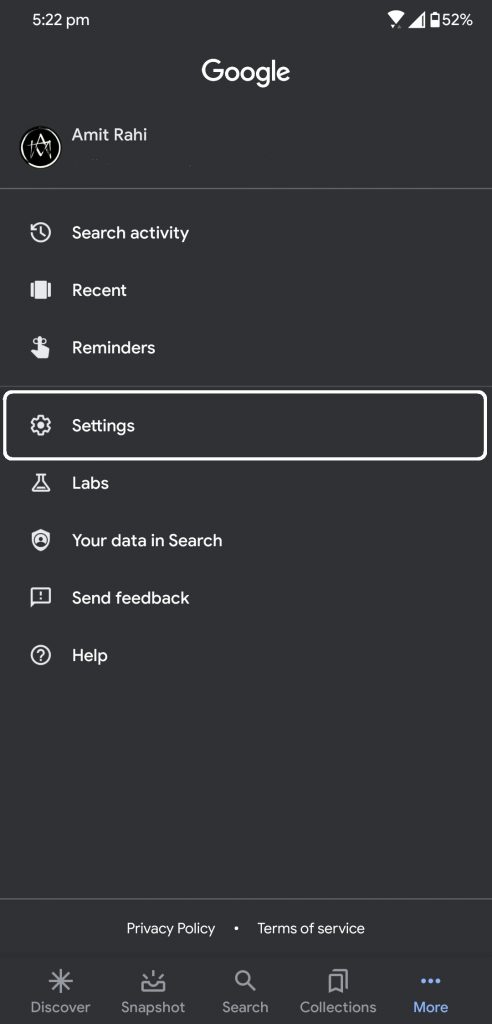The screenshot shows a Google search interface on a mobile phone at 5:22 PM, with a Wi-Fi connection and 52% battery remaining. The background is a dark slate gray, and the text is primarily white, with some elements in gray and blue. 

At the top, "Google" is prominently displayed in the center. Below it, the text "MIT" is followed by "RA", with these letters placed on the left side. Beneath this, a line separates the section from the options below, which include "Search," "Activity," "Recent," "Reminders," "Settings" (highlighted with a white rectangle), "Labs," "Your Data in Search," "Send Feedback," and "Help."

Further down, another line separates the main body from the footer section, which contains "Privacy Policy" and "Terms of Service." Below this, additional options such as "Discover," "Snapshot," "Search," "Connections," and an icon with three horizontal dots labeled "More" (in blue) are aligned horizontally.

On the left, there is a profile picture depicted as a geometric design in gray, set against a black background and encircled by a white border.

Overall, the interface features a dark gray background with white text and accents of gray and blue.